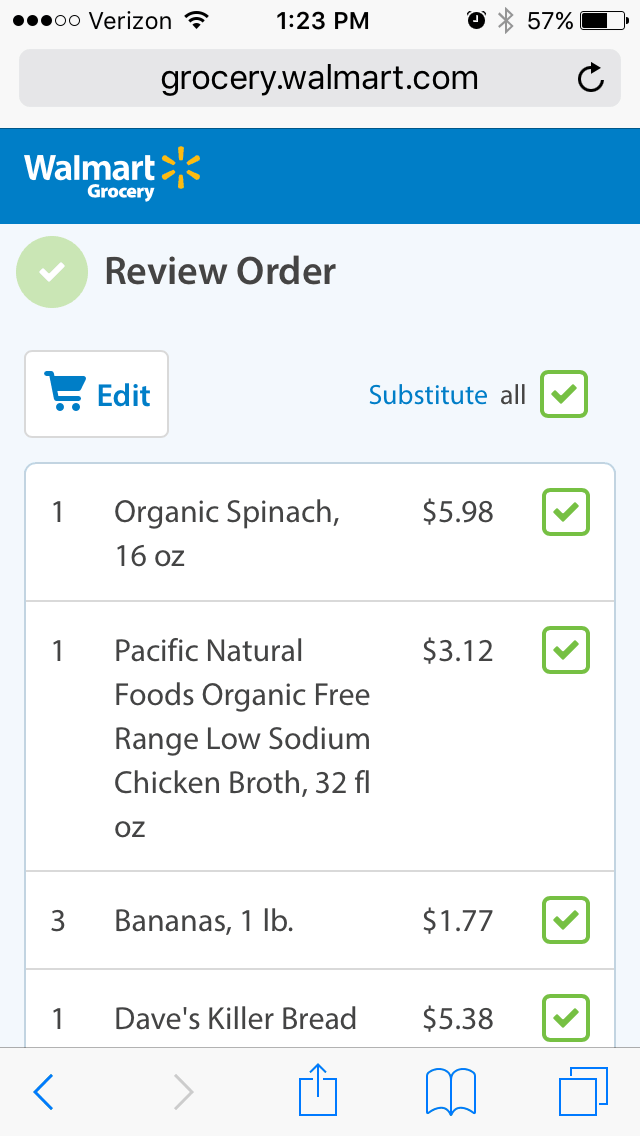A detailed screenshot showcases the Walmart mobile website on a Verizon mobile device. The time displayed is 1:23 PM with a battery life of 57%. Notifications indicate that both the alarm clock and Bluetooth features are active. The top left corner of the screen features the Walmart grocery icon prominently placed on a blue navigation bar. The currently visible webpage is the 'Review Order' page, which includes functions such as a shopping cart and an 'edit' button.
 
The order list includes:
- Organic Spinach, 16 ounces
- Pacific Natural Food, Organic Free Range, Low Sodium Chicken Broth, 32 fluid ounces
- Bananas, 1 pound
- Dave's Killer Bread priced at $5.38.

Each item is accompanied by a green check box housed within a green box, indicating its inclusion in the order. At the bottom of the screen, there are backward and forward browser navigation buttons, a bookmark button, and a share icon, providing additional user functionalities.